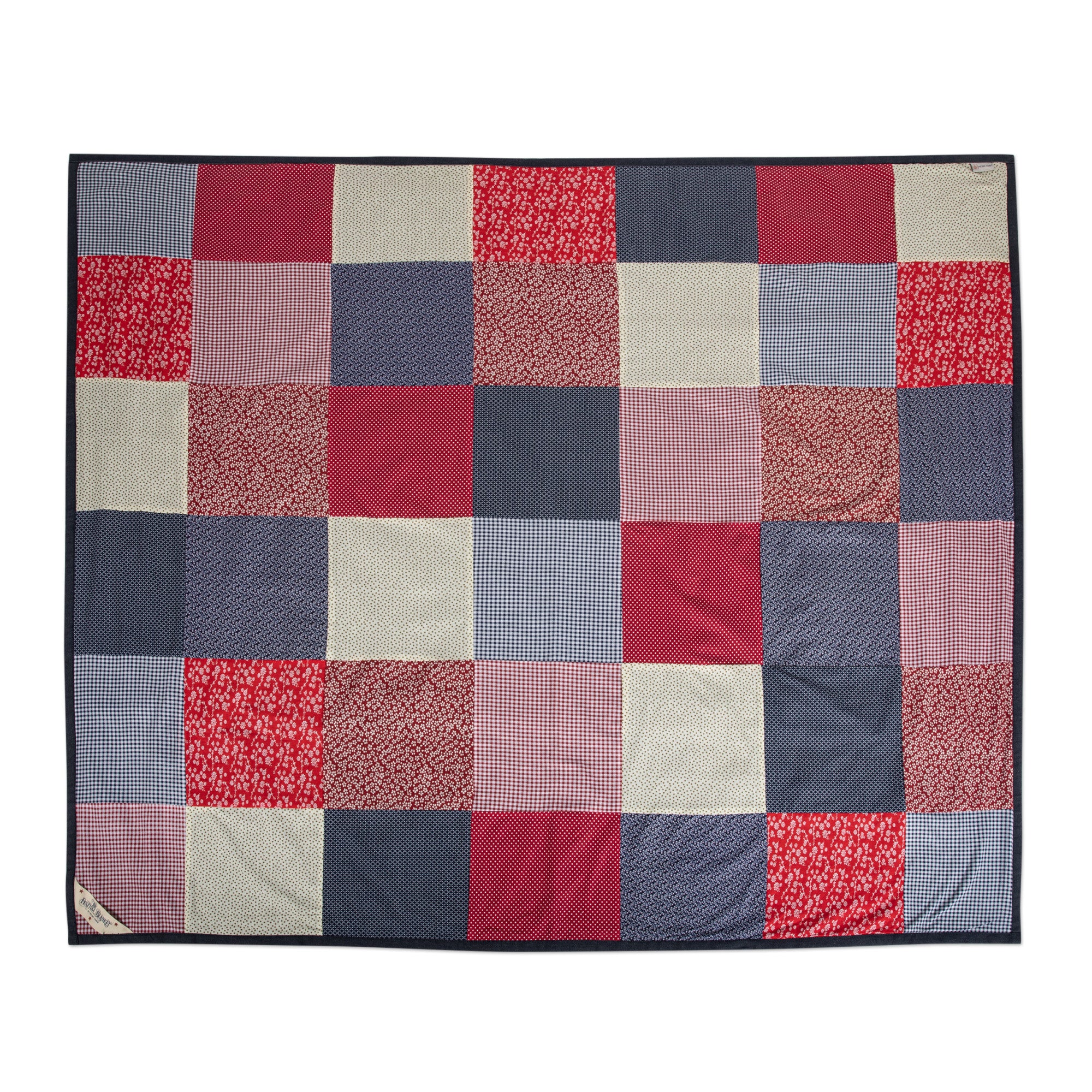This image showcases a rectangular quilt, meticulously crafted from an array of fabric squares sewn together. Each square varies in color and pattern, contributing to a cohesive yet random patchwork design. Noted prominently are patterns such as red and white gingham checks, blue and white gingham checks, and a variety of darker blues and beige hues. The quilt encompasses a broader color palette with an overarching theme of blue, white, and red, imparting an Americana feel.

The edging of the quilt is black, resembling a bias strip that runs along the perimeter. Situated in the left bottom corner, a small tag can be spotted. Despite the variety in patterns, which include intricate florals, simple plaids, and other calico designs, there doesn’t appear to be any decorative quilting stitching on the quilt's surface. A tiny tear is visible in the upper right corner. Estimating the composition, the quilt likely consists of around 42 squares, arranged in a 6x7 grid.